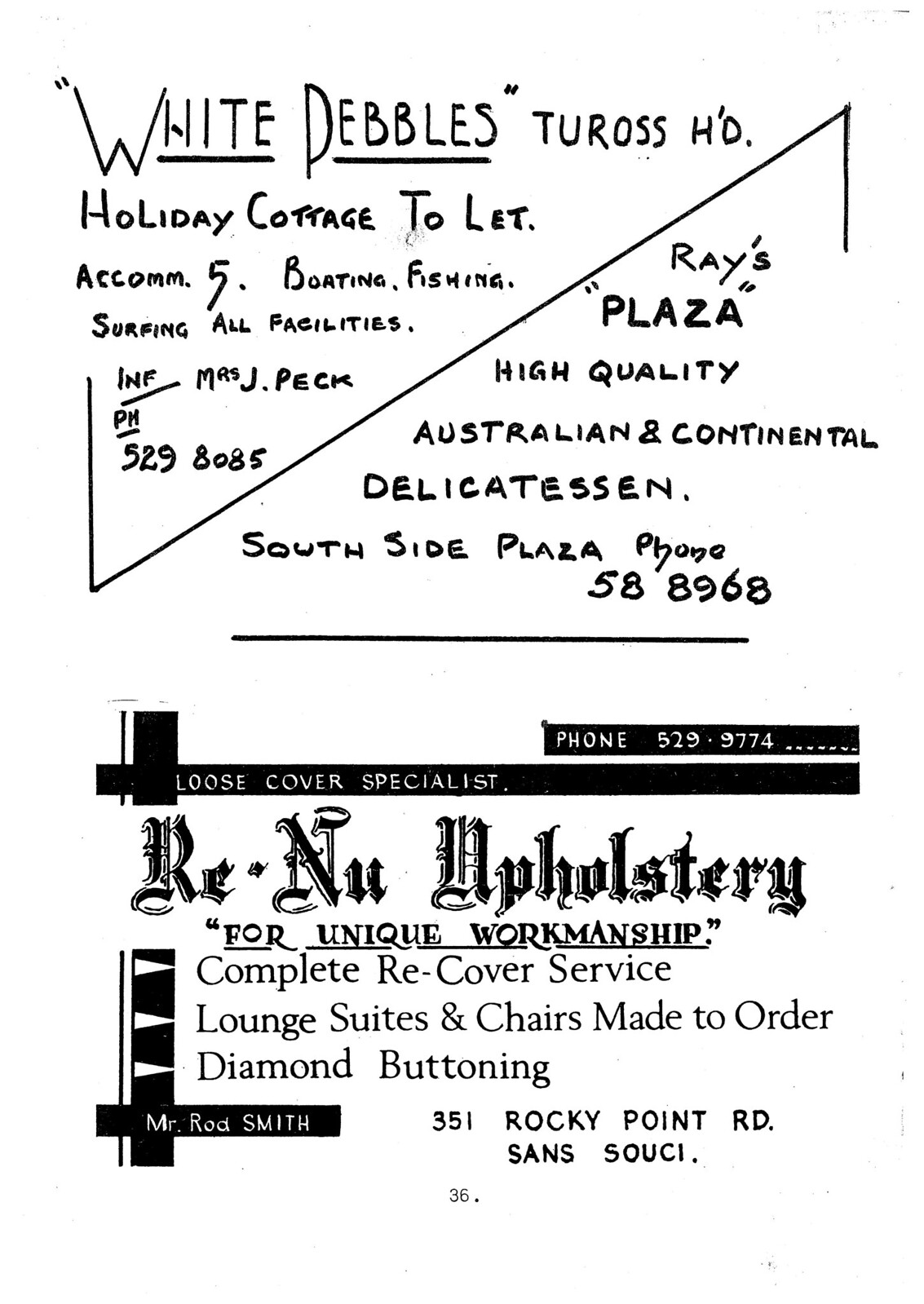This image, in portrait layout, features a white background with black text divided into two sections. The top section is divided further by a diagonal line. The top left quadrant appears hand-drawn and has text reading: "White Pebbles, Turas HD, Holiday Cottage to let, accommodates five, Boating, Fishing, Surfing, All Facilities, INF Mrs. J. Peck," followed by a phone number. On the bottom right of this section, it reads: "Ray's Plaza, High Quality Australian and Continental Delicatessen, Southside Plaza," with another phone number beneath it.

The bottom half of the image has a more professional and high-quality print design. It includes a black bar at the top with white text showing a phone number, followed by another black bar stating "Loose Cover Specialist". Below this, black font outlines the services: "Renew Upholstery for Unique Workmanship, Complete Recover Service, Lounge Suites and Chairs Made to Order, Diamond Buttoning," accompanied by an address and the name "Mr. Rod Smith". This appears to be a collection of different advertisements, possibly from a local zine or community bulletin.